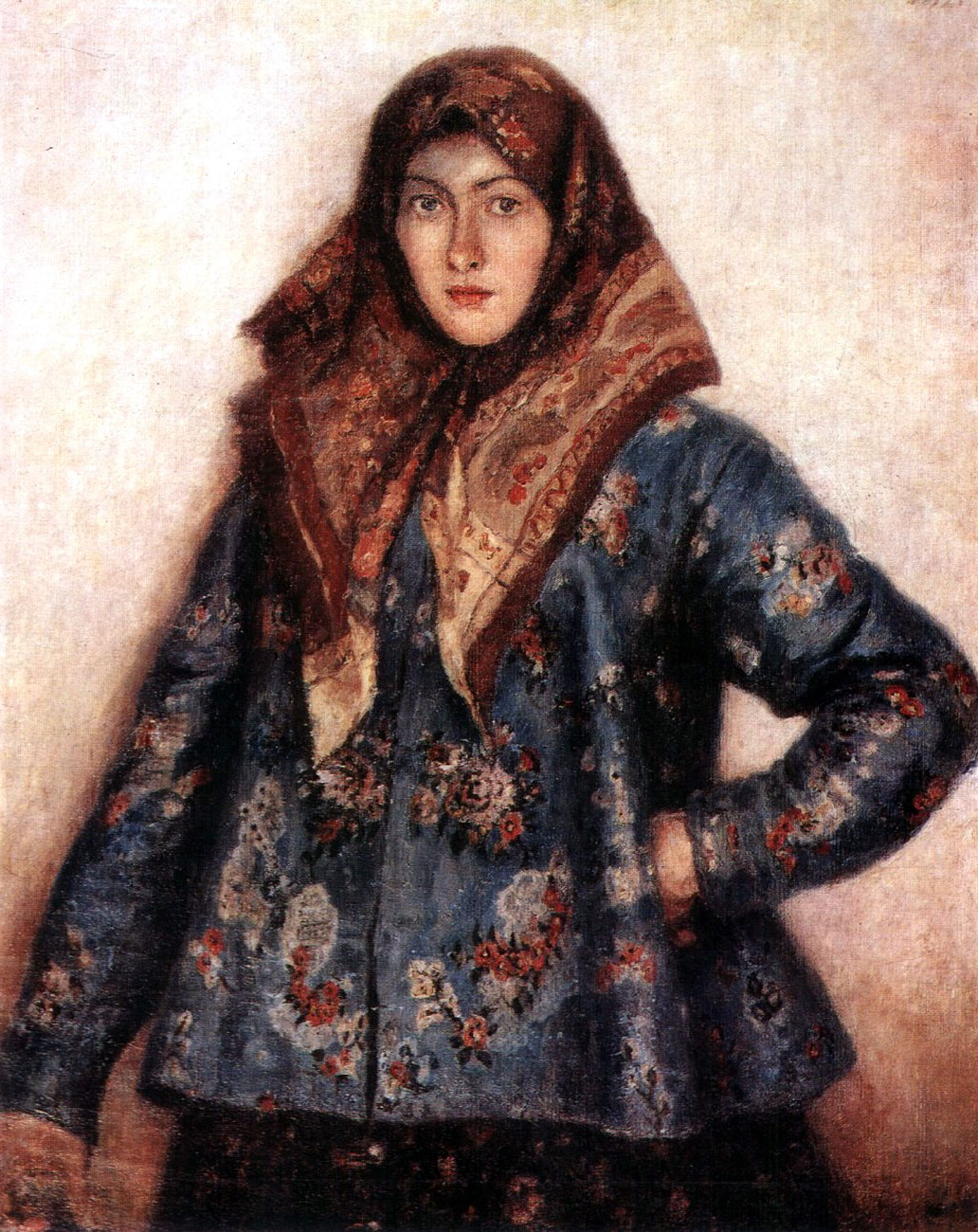This is a highly detailed portrait painting of a young white woman, likely in her 20s or 30s, depicted indoors. The background is a light, neutral shade, ranging from beige to taupe with pinkish and mauve undertones, resembling a softly lit wall. The woman stands confidently, looking straight ahead with a composed, straight-faced expression.

She has striking red lips and dark eyebrows that frame her face, along with a distinctive long nose. She wears an elaborate headscarf with a complex pattern, dominated by black, red, and brown hues, featuring floral and paisley designs. The headscarf is artfully draped around her head, tucking under her chin and extending downwards to form long triangle shapes in front of her chest.

Her attire includes a very elaborate and flowy blue jacket adorned with an intricate floral print in shades of red, white, and possibly copper. The jacket has an ornate design, giving it a shiny, luxurious feel. Her left hand rests in a fist against her hip, creating a triangular shape, while her right arm hangs straight down by her side. She also wears a black skirt, and the painting captures her from the upper thigh up.

The overall composition highlights both the intricacy of her clothing and the serene, poised demeanor of the woman against the softly colored backdrop.